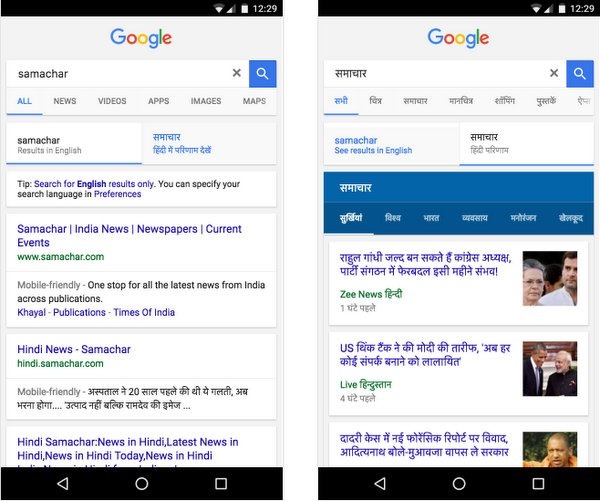The image is horizontally rectangular and features two side-by-side screenshots of cell phones displaying the Google search page. Both screenshots showcase the familiar Google logo at the top, followed by the search field. Below the search field are the various search categories: All, News, Videos, Apps, Images, and Maps.

On the left phone, the search query entered is "Samachar" (S-A-M-A-C-H-A-R), whereas the right phone displays a search query in another language. Despite the language difference, both results are translations offering the same news stories. The left phone's Google page includes a tip stating: "Search for English results only. You can specify your search languages and preferences."

The search results for "Samachar" are displayed below the navigation options. The first result on the left phone reads "Samachar - Indian News, Newspapers, Current Events" from samachar.com. The second result is "Hindi News Samachar" from hindi.samachar.com. The right phone, showing the same news in a different language, indicates how Google translates and provides parallel information across different languages.